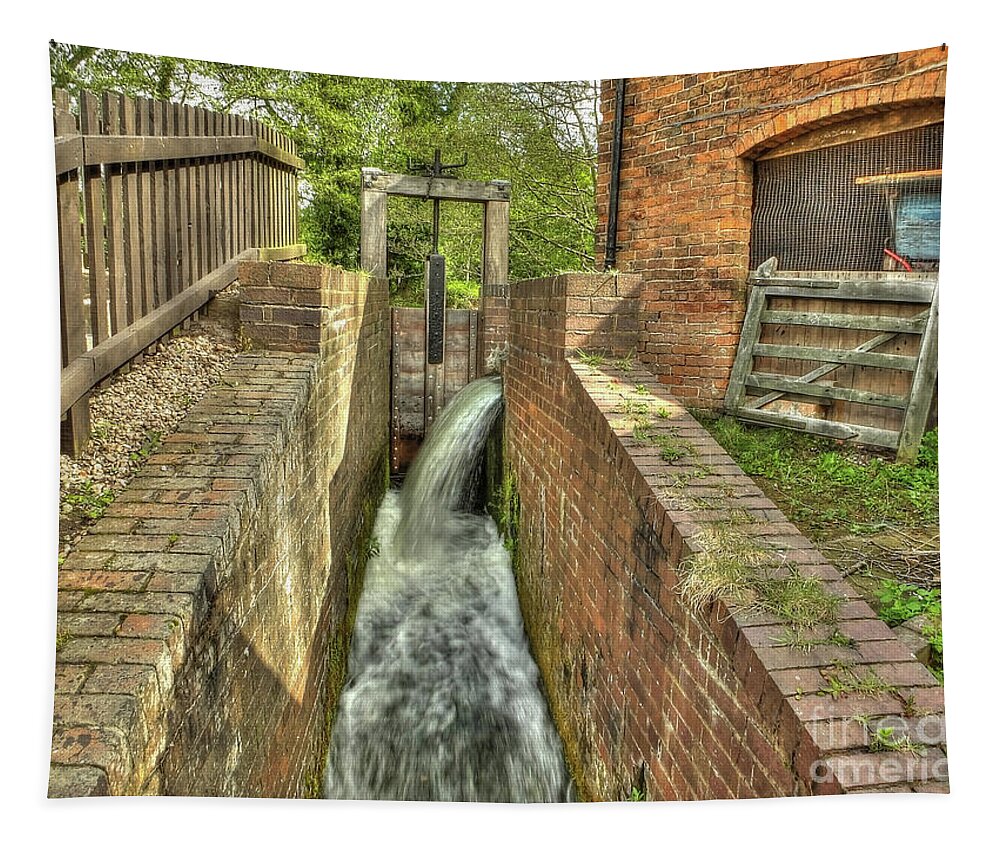The photo depicts a narrow, deep water channel, surrounded by high brick walls, likely part of an old water management facility or possibly a historic structure like an old asylum or castle. The foreground showcases water flowing from an unseen gate, creating a small waterfall into the channel below. On the left side, a wooden fence can be seen, framing the scene, with a wooden pallet or section of a fence leaning against a nearby brick building. This building, partially obscured, features a distinct U-shaped, wooden frame structure. In the background, behind the sluice gate system, a North American deciduous forest adds a touch of natural beauty to the otherwise industrial and historical setting.